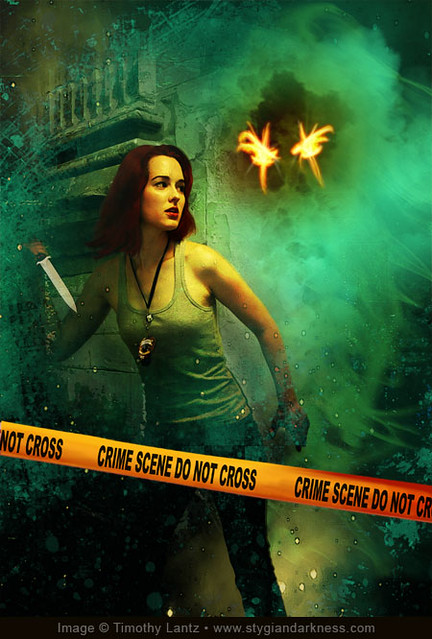The image depicts a digitally created scene featuring a woman with short dark hair and a lighter skin complexion, clad in a gray tank top and dark pants. She holds a knife in her hand, poised in an aggressive stance, looking to her right. A spectral figure or spirit, emerging from a plume of green smoke, looms behind her with ominous, glowing eyes. The entire scene is accentuated with faded concrete block patterns and scattered green splotches. Yellow-orange police tape, emblazoned with the words "Crime Scene Do Not Cross" in black letters, stretches across the lower half of the image. At the very bottom, there's a credit line reading "Image Timothy Lance" followed by the website "www.stygiandarkness.com."